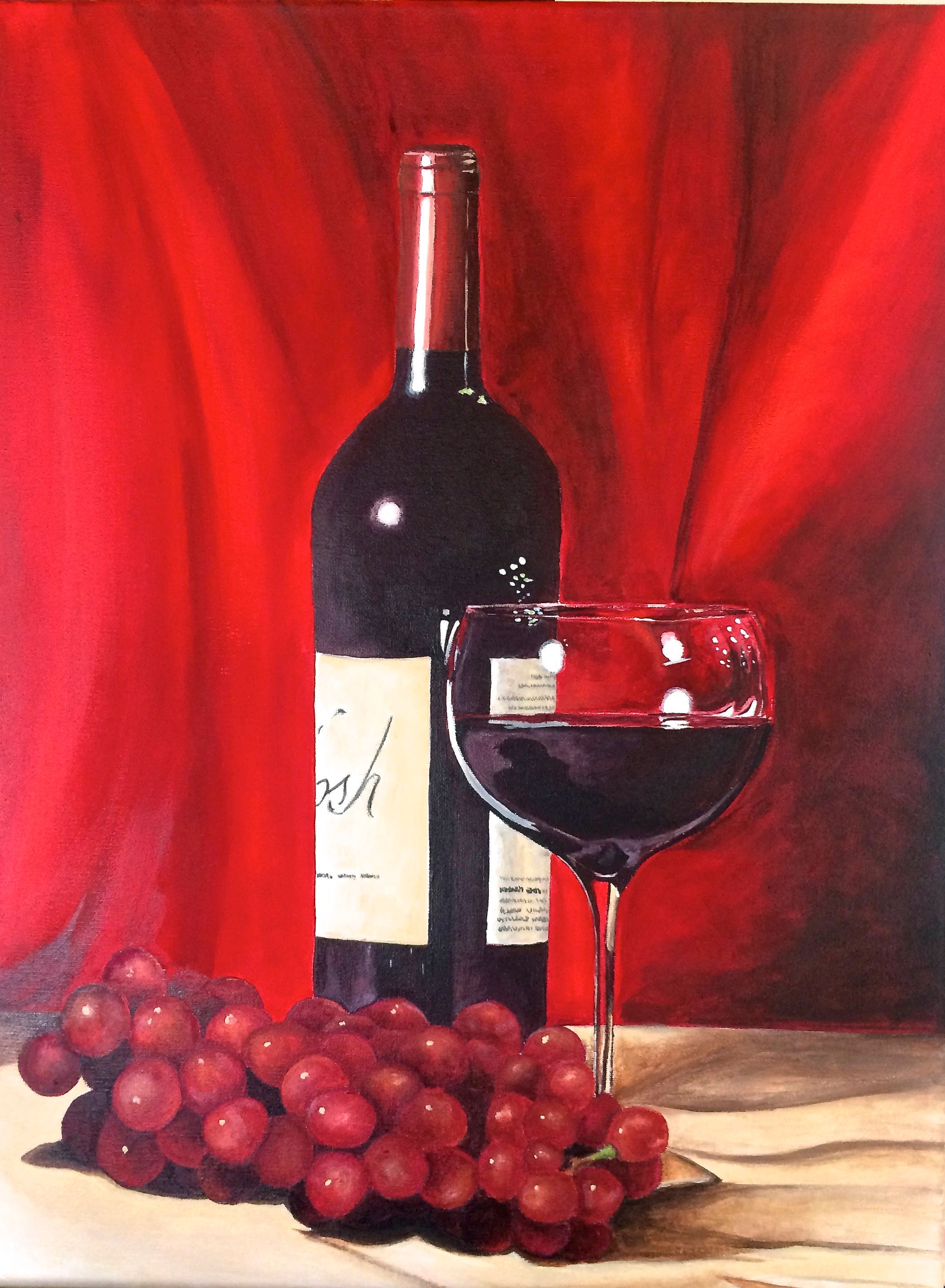The still life oil painting captures a serene and elegant scene featuring various elements associated with wine. Central to the composition is a bottle of red wine, slightly turned so that its label is obscured, with a half-filled wine glass positioned to its right. Both the bottle and glass rest on a light tan tablecloth draped over a table, contrasting beautifully with the rich red curtain in the background, which might sometimes appear like a red wall due to its texture and depth. Sprawled in front of the bottle and glass is a vine bearing plump red grapes, which stretches from the left to the right, suggesting the origin of the wine. The meticulous details and realistic quality of the painting initially give the impression of a photograph, capturing the depth of shadows and the subtle interplay of light on the objects, adding to the illusion of reality.